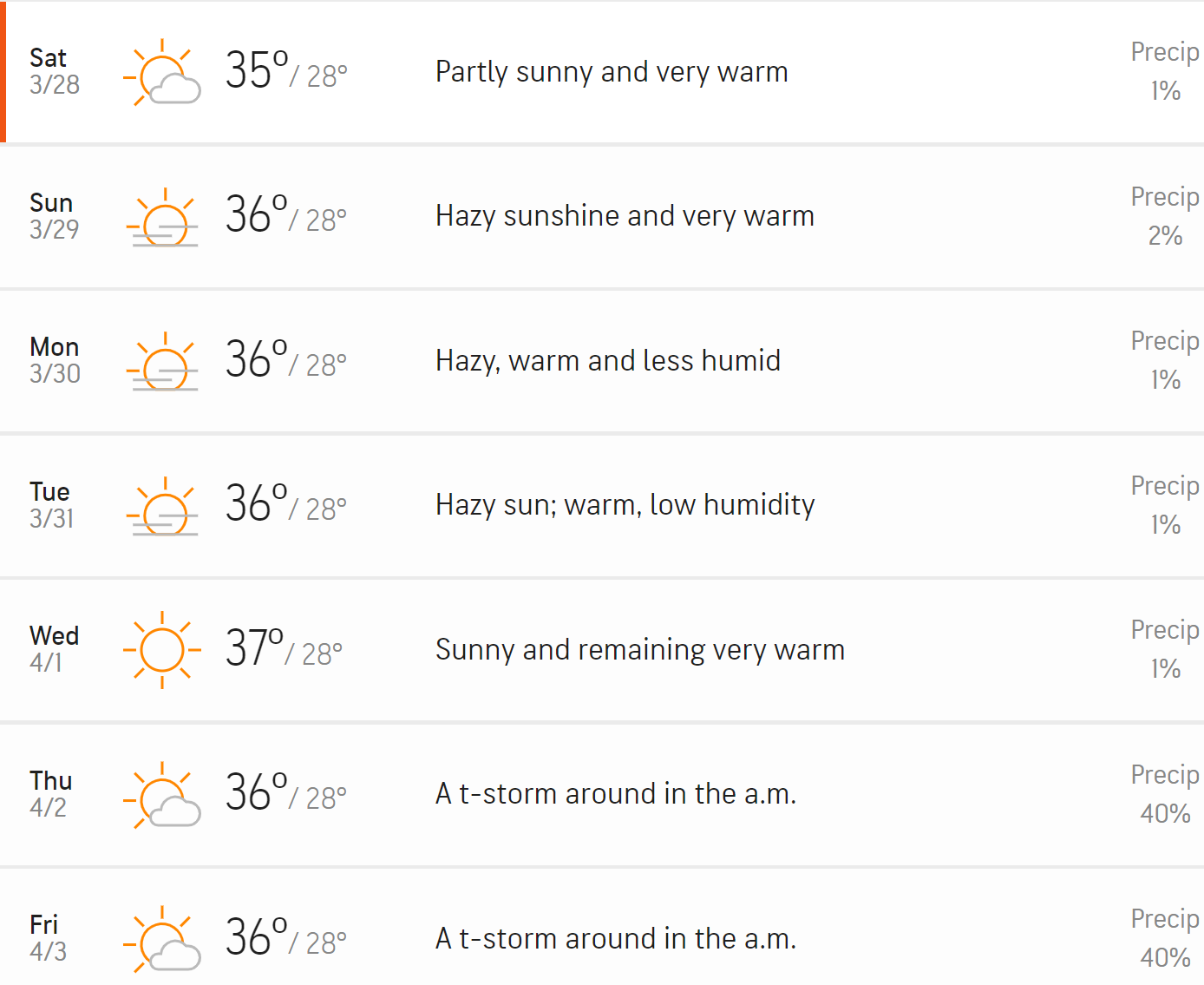A detailed weekly weather forecast is illustrated, spanning from Saturday, March 28th to Friday, April 3rd.

- **Saturday, March 28th:** At the top is the day “Saturday” in bold, followed by the date "3/28" in a light gray text. To the right, there's a small icon showing a sun partially covered by a gray cloud, indicating partly sunny weather. The high temperature, prominently displayed, is 35°F, with a low of 20°F in smaller text. Below, there's a brief description: “Partly sunny, very warm.” The precipitation chance is listed as 1%.

- **Sunday, March 29th:** Here, "Sunday" is bold with "3/29" beneath it. The weather icon appears to depict the sun with a line through it, which likely represents hazy sunshine or windy conditions. The high is 36°F, with a low of 28°F. The description reads: "Hazy sunshine, very warm.” Precipitation is at 2%.

The layout continues similarly for each day of the week, providing a concise but clear presentation of daily weather conditions. Each day’s forecast includes:
- The day of the week and date at the top.
- An emoji indicating the general weather.
- Bolded high and low temperatures.
- A brief descriptive phrase summarizing the weather conditions.
- A column on the right with the day’s precipitation percentage.

This format repeats, ensuring a consistent and easy-to-understand presentation for the entire week.